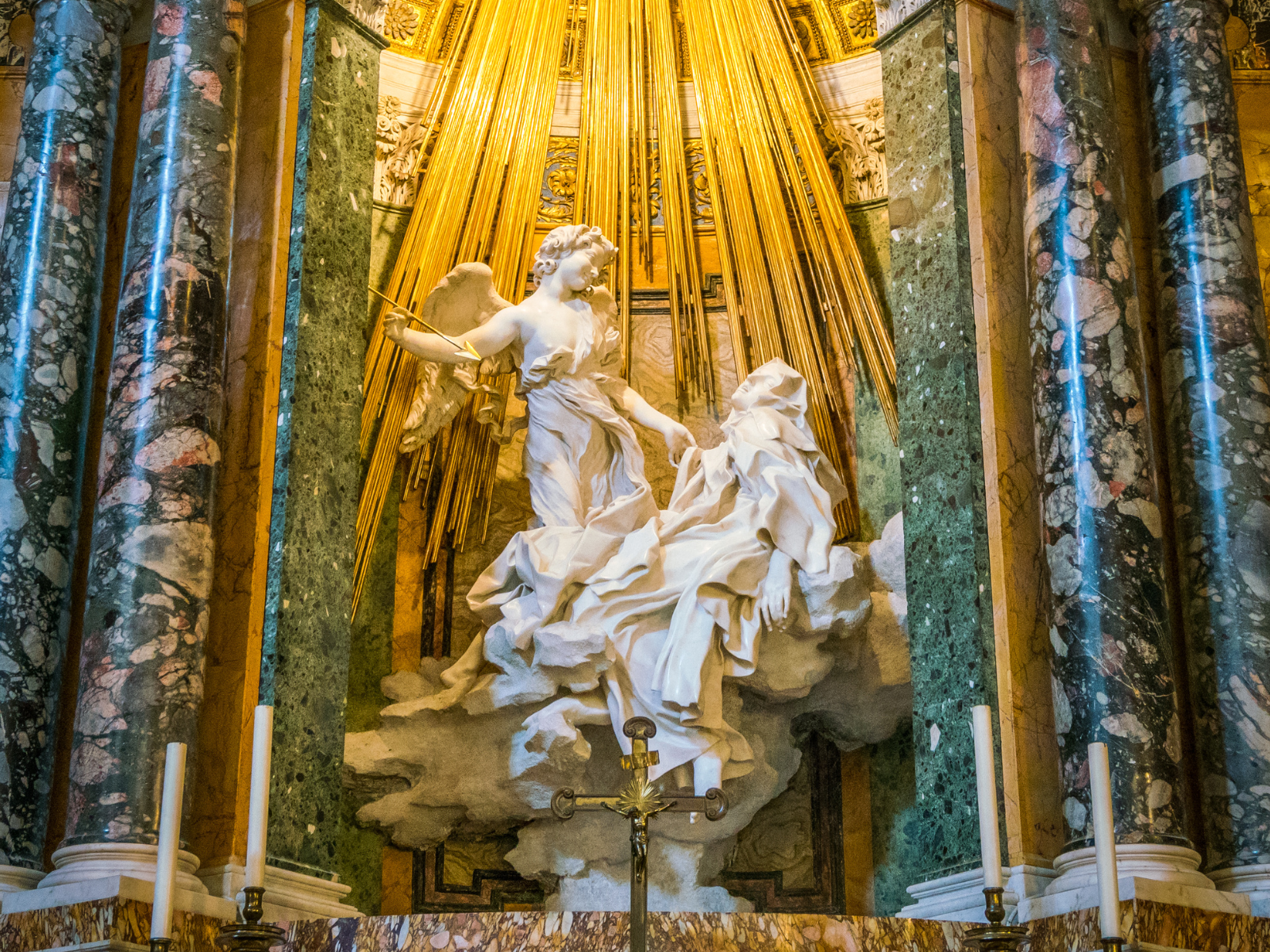This photorealistic image captures an intricate religious display within a cathedral or church, characterized by its elaborate design and marble columns flanking the scene. At the center is a striking statue featuring an angel wielding an arrow, poised to strike another figure dressed in flowing robes, likely representing Jesus. The setting includes an altar and a pair of candles situated near the pillars. Above and behind the statues, golden lines or strands hang down, augmenting the old-style church aesthetic. The photograph is taken from a low angle, allowing a view of the decorated ceiling and enhancing the grandeur and sacred ambiance of the place.